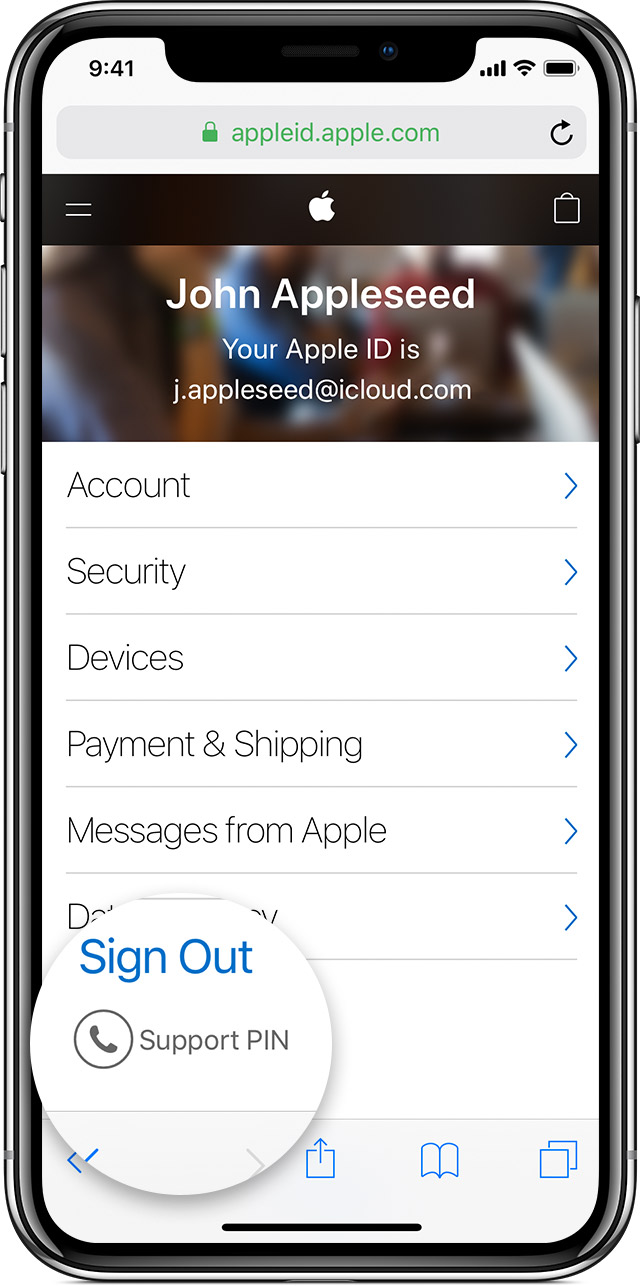The vertically-oriented image features a smartphone positioned against a white background, which is actually illuminated by a computer screen. The smartphone has a sleek black rim that is slightly reflective. 

On the smartphone screen, the top left corner displays the time, "9:41 AM." On the top right corner, the icons indicate full signal strength, a strong Wi-Fi connection, and a fully charged battery.

Beneath these details, the website URL "appleid.apple.com" is shown in green text. Below the URL, a dull black navigation bar is visible. On the left side of the bar are two clickable lines (menu icon), in the center is the Apple logo, and on the right is a small bag icon, suggesting a shopping cart or store link.

The background beneath the navigation bar is purposefully blurred, yet it seems to depict a group of people or a crowded place. Centrally displayed on the screen is the name "John Appleseed," alongside the message "Your Apple ID is j.appleseed@icloud.com."

Further down, a white section lists various options: Account, Security, Devices, Payment & Shipping, and Messages from Apple. However, the last option is partially obscured by a pop-up circle, which includes the "Sign Out" option and a button labeled "Support PIN" along with some icons at the bottom of the screen.